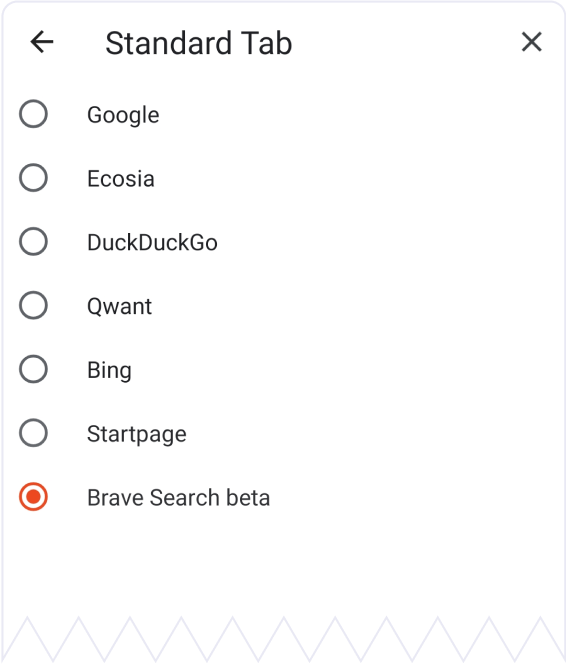The image depicts a user interface for selecting a default search engine from a list. The background is plain white. At the very top of the interface, there is a left-pointing arrow followed by the text "Standard Tab" in a large, dark font. In the top right corner, there is a prominent "X" icon. Below this header, there is a vertical list of search engine options, each with a round, hollow circle to the left that serves as a selection button.

The first option is "Google," followed by "Ecosia," "DuckDuckGo," and "Qwant." Continuing down the list, "Bing" has a hollow selection circle, similar to the previous options. Below "Bing" is "Startpage."

At the very bottom of the list, there is a unique red circle filled with a red dot in its center, indicating that the option "Brave Search Beta" is currently selected. The interface ends with a zigzag pattern cut across the bottom edge.